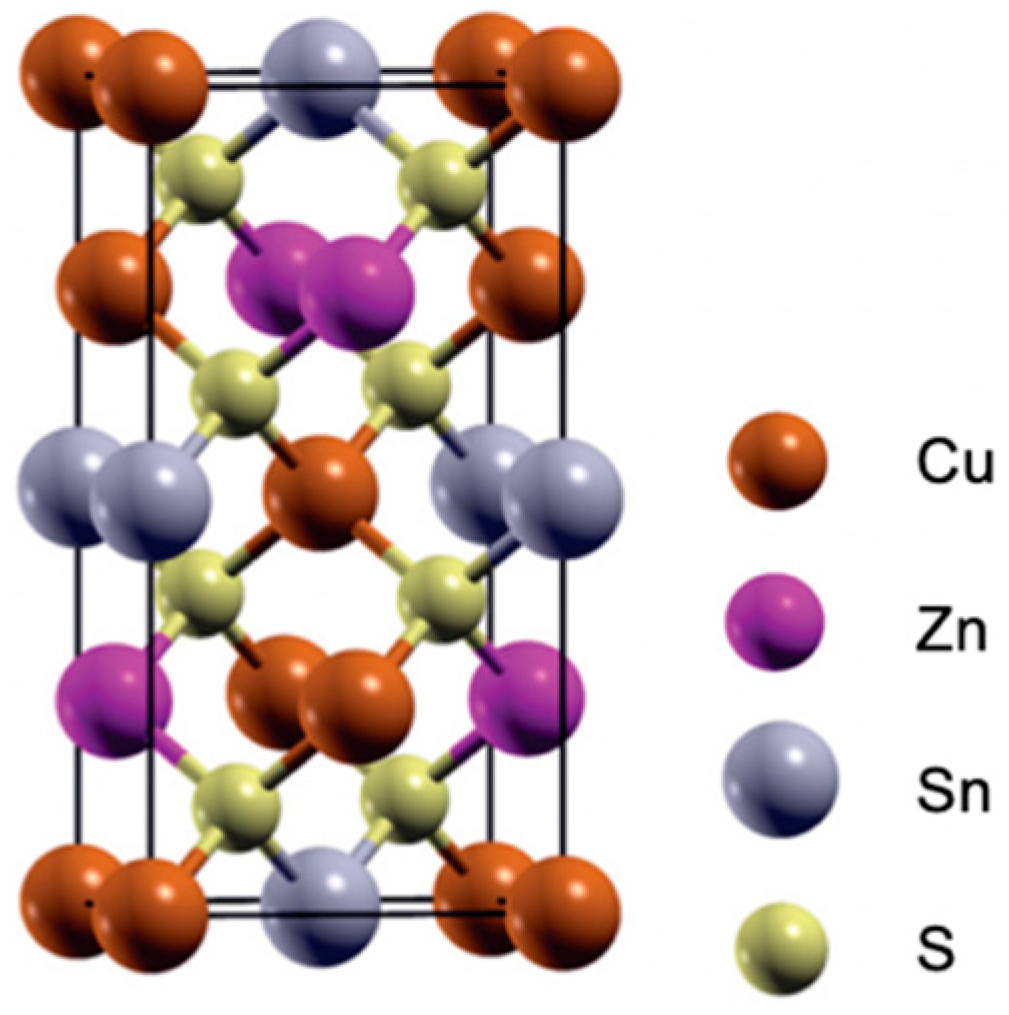The image appears to be a computer-generated rendering of a molecular structure, depicted through various colored spheres connected by black rectangular connectors. The spheres come in distinct colors, each corresponding to a specific element, as indicated by a color legend on the right side. The legend clarifies that orange spheres represent Cu (Copper), purple spheres represent Zn (Zinc), gray spheres represent Sn (Tin), and green spheres represent S (Sulfur). The molecular structure itself seems scientifically sound, with the spheres arranged and connected diagonally, although not in an exact pattern, suggesting a complex scientific representation of a molecule. The orange (Cu) and gray (Sn) spheres are prominently positioned at the top and bottom, while the green (S) and purple (Zn) spheres are interconnected throughout the structure, further emphasizing the detailed and intricate nature of the diagram.